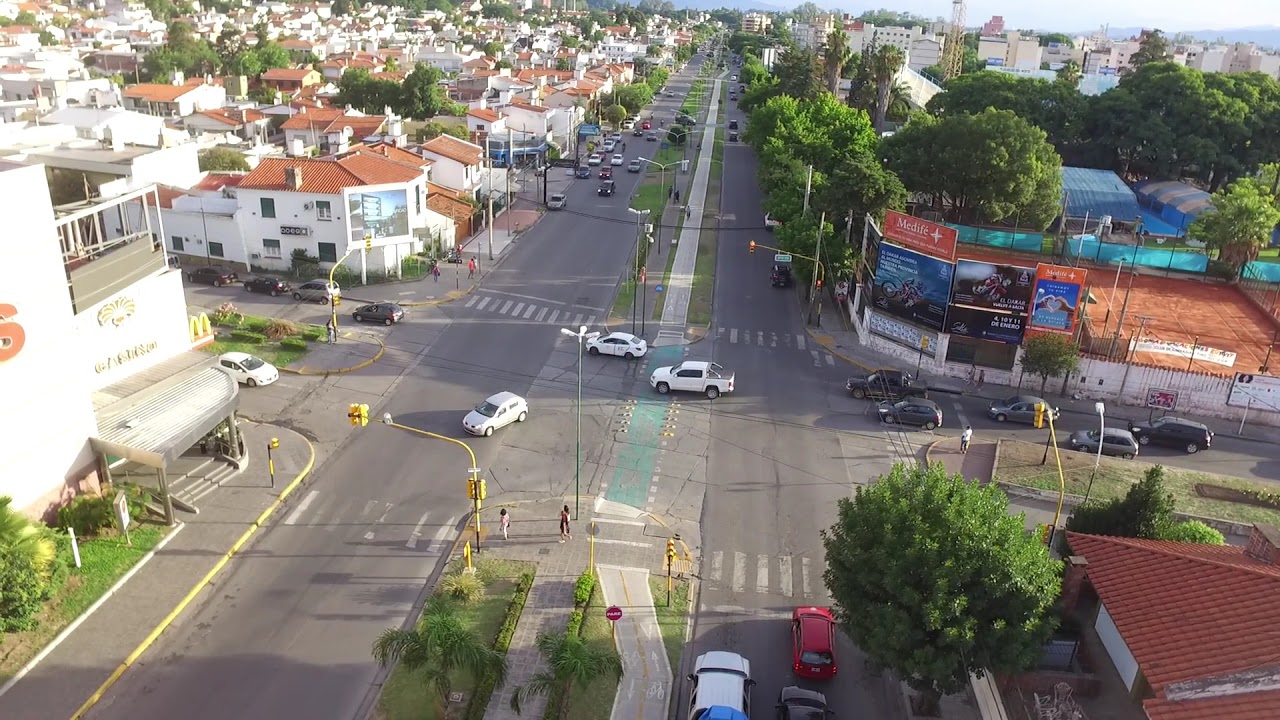This aerial image depicts a vibrant city intersection bathed in midday sunlight, revealing a detailed and colorful urban landscape. At the center of the image, a prominent roadway stretches vertically from the bottom to the top. Flanking this road on both sides are a mix of residential and commercial buildings, with various architectural styles and colors including green, brown, white, gray, yellow, red, orange, and blue. The clear image highlights streetlights and crosswalks, capturing a dynamic street scene with several people walking along the sidewalks and waiting at crosswalks. The road appears flanked by both homes and businesses, with cars dotting the streets and parked along the curbs. Additionally, the image features a notable walking trail running parallel to the main roadway, suggesting it could be a repurposed rail line, discernible from the unique layout and markings at intersections. The scene is devoid of any readable text or numbers, emphasizing the purely visual narrative of a bustling city during the day.